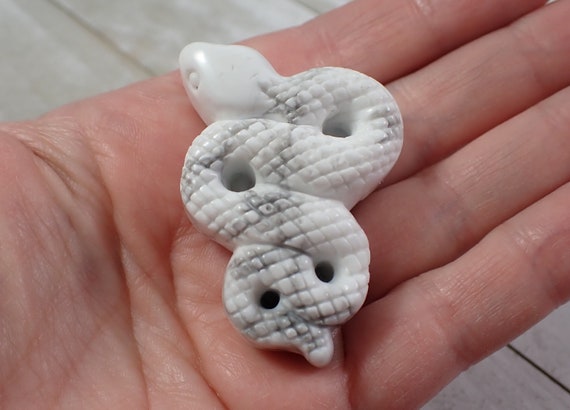In this detailed color photograph, a man's left hand emerges from the lower left corner, with his palm open and fingers extending towards the upper right. Resting on his palm is a small, intricately carved stone sculpture of a snake. The snake sculpture is crafted from white and gray stone, giving it a patterned appearance that resembles the natural scaling of a real snake. The snake is curled in a spiral, reminiscent of an ice cone shape, with its smooth white head pointing upwards and slightly to the right. The body of the snake features subtle black highlights, adding to its lifelike appearance. The statue is approximately the width of the human hand holding it, with the detailed carving capturing the delicate texture and pattern of a snake's scales. Four small holes are visible on the snake's patterned body, two larger and two smaller, further emphasizing the detailed craftsmanship of this petite, stone-carved serpent.